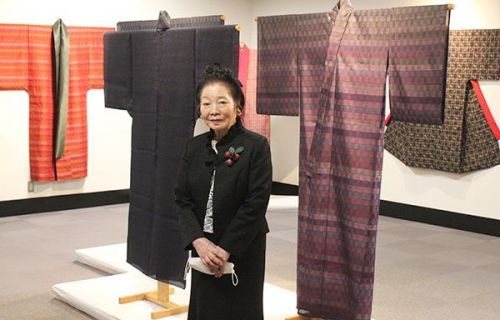This detailed color photograph, taken in landscape orientation, depicts an older Asian woman, likely in her 70s or 80s, standing in the center of a museum setting that appears to focus on kimonos. She has black hair tied neatly back in a bun and is dressed formally in a black suit jacket adorned with a plum brooch on the lapel, a white shirt underneath, and a black skirt. Her hands are folded in front of her waist, holding a white clutch bag and possibly a face mask.

The museum background features several displays of kimonos, held up on wooden stands and attached to walls, creating a layered, textured backdrop. The kimonos exhibit a range of colors and patterns, including black, purple horizontal stripes, and an orange horizontal stripe. Specific fabrics display deep purple, light purple, yellow stripes, and some silky textures. The walls of the museum are white with black baseboards, and the floor is tiled in varying shades of gray. The photograph captures a blend of representationalism and realism, with the woman making eye contact with a half-smile, inviting the viewer to engage with the cultural and artistic richness of the setting.